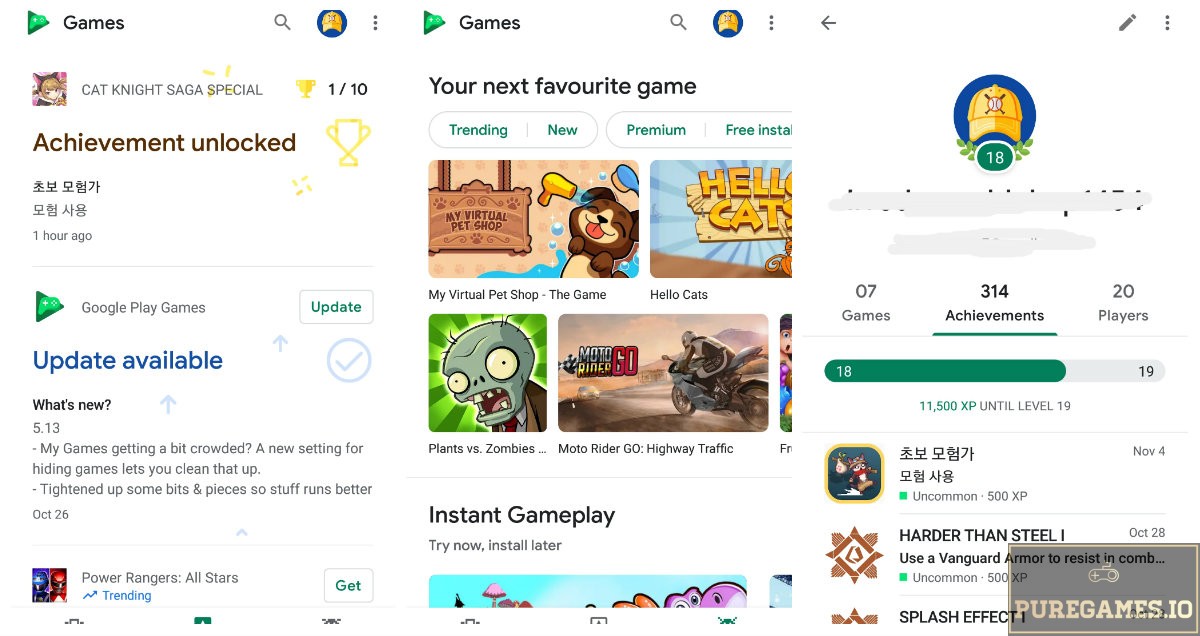**Detailed Caption:**

The webpage is divided into several sections with different icons and text elements. In the upper left-hand corner, there is a green play symbol resembling a sideways arrow, overlayed with a lighter gray icon. To its right, the word "Games" is displayed, followed by a black magnifying glass icon representing the search function. Next to the search icon, there is a blue circle with a yellow baseball cap inside. To the right of this are three vertically aligned black dots, indicating a menu. Another green play symbol with a green icon is placed next to these dots, followed by the word "Games" inside a search bar. Moving further right, there’s another search icon, the blue circle with the yellow baseball cap, and another three vertical dots. A black left-pointing arrow is situated to the right of these elements, and to the right of that is a black pencil icon followed by another set of three vertical dots.

Beneath this toolbar, there is a pink box featuring a blonde anime girl. To the right of this image, "Cat Knight Saga Special" is written in black, with "Knight" spelled as K-N-I-G-H-T. Further right, there is a gold trophy icon and the text "1/10" in black. Below this is a bold black heading that reads "Your Next Favorite Game," and adjacent to it is a larger blue circle containing a yellow baseball cap, positioned above a green circle with the number 18 in white.

On the left-hand side of the page, under the "Cat Knight Saga" title, the phrase "Achievement Unlocked" is written in brown, accompanied by a gold trophy icon. Below this, two rows of Asian characters are displayed, followed by the text "1 hour ago" in black. Nearby is the green arrow logo with the text "Google Play Games" beside it, and across from it is a white bar with "Update" written in green. Below this, in blue text, is an "Update Available" notification, followed by "What's New," and the version number "5.13." Subsequent text reads: "My game's getting a bit crowded? A new setting for hiding games that you…" Below that, another line reads: "Tightened up some bits and pieces so stuff runs better."

Directly under the "Your Next Favorite Game" heading, there are white bars with green text labels: "Trending," "New," "Premium," and "Free Install," though the latter gets cut off. Below these categories, an image of a brown puppy is displayed with a wooden sign to its left that says "My Virtual Pet Shop." Next to this image, there is another picture with part of the text visible, showing "Hell" and "Cats" on a wooden sign. This is followed by an image of a green zombie in a brown suit and another image of a man riding a motorcycle, captioned "Motor Rider" with "Go" written in red. "Instant Gameplay" is written in black beneath this section.

On the right-hand side, a blue circle with a yellow baseball cap icon is shown, with the text "0.7 Games" beside it. Below that, "3.14 Achievements" is underlined, followed by "20 Players." Below this, a bar graph is half green, half yellow, and gray, with the number 18 in white on both ends but with a variance, as it displays 19 in black on the right side.